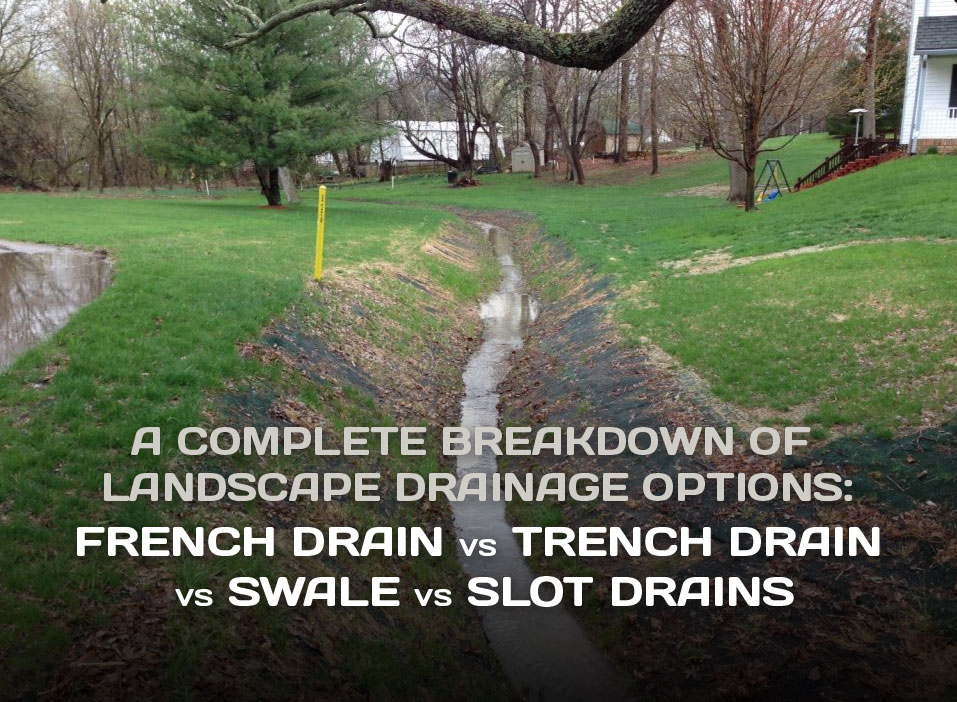This horizontal rectangular image captures a scenic view of a landscaped yard. In large gray letters at the bottom, two lines of text read: "A complete breakdown of landscape drainage options," with larger white letters below stating: "French drain versus trench drain versus swale versus slot drains." The image reveals a white house perched at the top of a hill, surrounded by lush greenery. The land slopes downward on either side, converging into a shallow ditch that seems to have once been paved with asphalt or cement, now overgrown with moss and grass. A gentle stream of water flows down the center of this trench, winding between the house and an adjacent property, before curving away towards the background. To the left of the ditch is a possible flooded area or pond. The yard is framed by deciduous trees and a few pine trees, creating a picturesque backdrop. On the right side, a white house with descending stairs is visible, along with additional lawn space. The scene is complemented by a smaller shed with a green roof near the background, contributing to the serene and well-maintained landscape.